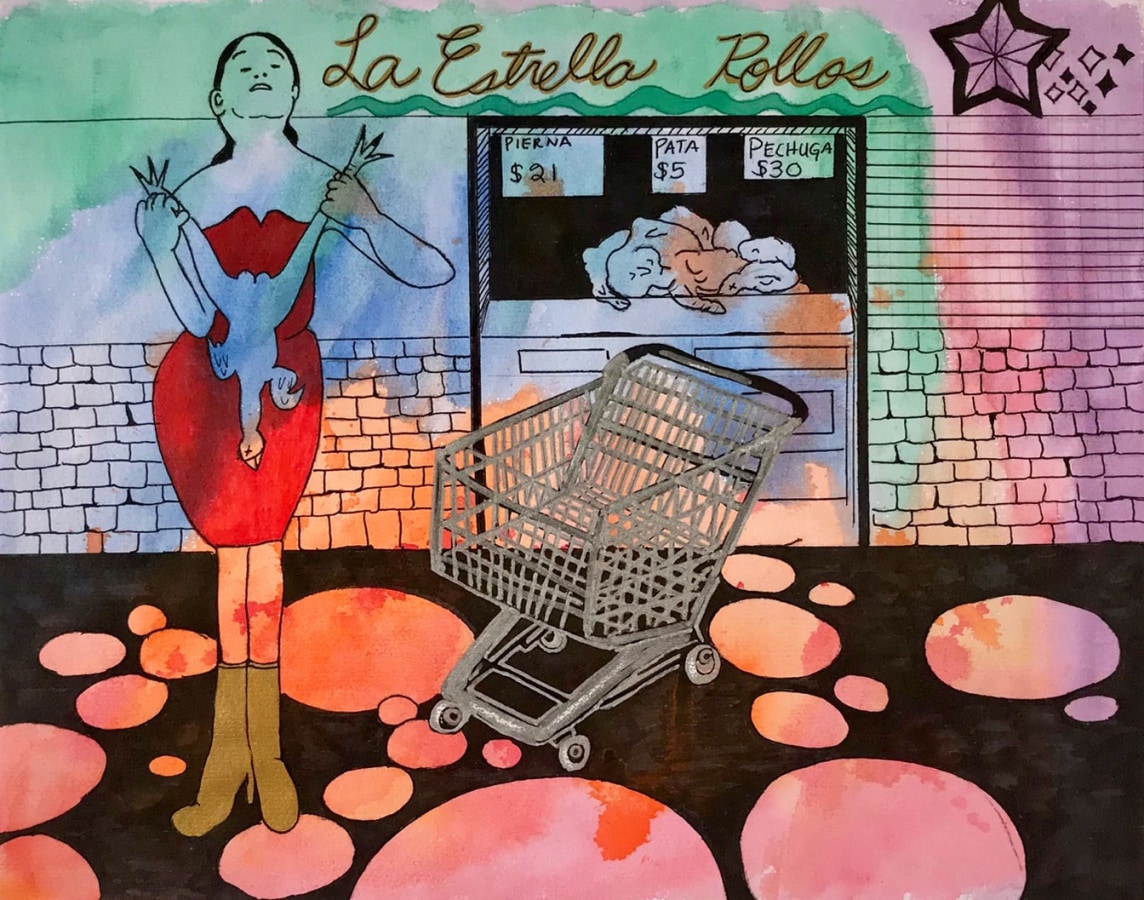In the image, titled "La Estrella Rolos" in cursive script at the top, a central black-bordered star is flanked by eight diamonds—four shaded black and four uncolored. Below this, three Spanish signs provide prices for various cuts of meat: "Pierna" at $21, "Pata" at $5, and "Pechuga" at $30. A bustling scene unfolds in front of a deli counter, where a woman, donned in a form-fitting, strapless red dress that reaches her knees and brown boots, holds an upside-down chicken by its legs. She stands on a black floor adorned with large red circles of varying sizes. A silver shopping cart with a black handle is angled beside her, adding to the sense of movement. The backdrop is a blend of green, blue, and pink watercolor, depicting a brick wall with horizontal stripes. The woman, sketched in black and white along with the chicken and bricks, contrasts with the colorful environment, creating a striking mixed-media composition.